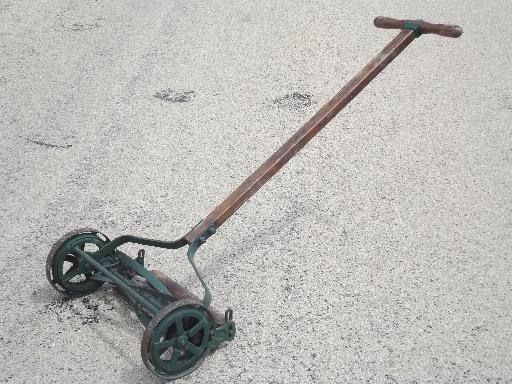This image depicts a well-used, old-fashioned manual lawnmower laying flat on a white sandy surface. The lawnmower features a long wooden handle with a horizontal, bar-like handlebar at the top for pushing. Its shaft leads down to a metal frame painted in a worn hunter green, attaching two circular wheels. A crossbar connects the wheels, and a series of six spinning blades are designed to cut grass as the mower is pushed forward. The paint around the wheels and the overall appearance indicate significant wear and use. The white, off-white sandy ground highlights the mower’s age and traditional design.